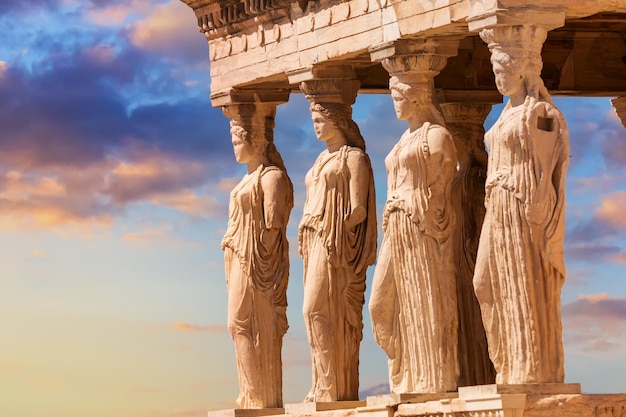This photo, taken outdoors during the day, captures an ancient structure featuring four intricately sculpted female statues acting as pillars beneath a top level, reminiscent of classical Greek architecture. These stone statues are carved to resemble women, each with a unique condition regarding their arms: the first statue has no arms, the second has shoulders but no full arms, and the remaining two have arms up to their elbows. The statues, dressed in long, cape-like garments, are standing side-by-side and all are facing toward the left side of the frame. Above these statues is a rectangular section of the structure. The color of the statues appears to be in earthy tones, ranging from clay to white. In the background, the sky features clouds with nuances of bluish purple and white, adding depth to the historic and serene atmosphere of the image.